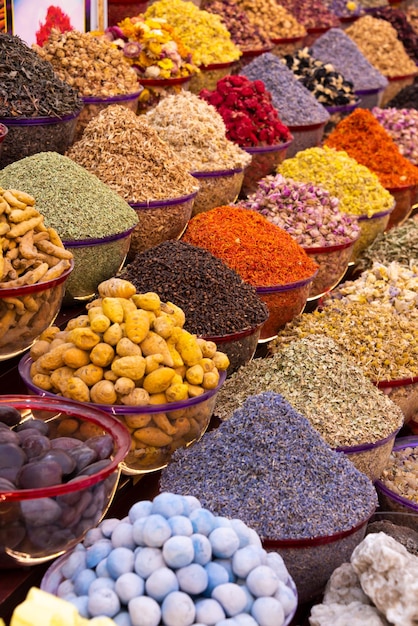This is a vibrant photograph taken outdoors during the daytime, showcasing a bustling spice market. The image captures five rows of round, clear containers piled high with a variety of colorful spices, fruits, grains, and roots. The rows are arranged ascending from the lower left to the upper right, creating a stair-like effect. Each container features a colored rim, adding to the vivid display. The assortment includes greens, browns, reds, yellows, purples, and grays. Notable items include ginger, garlic, light blue plums, various potatoes, and what looks like turmeric, spring onions, saffron, and grapes. Some containers are filled to the point of forming small pyramids above the bowls, adding to the market's bustling atmosphere. The background becomes blurrier towards the back, making it challenging to distinguish the contents of the farthest rows. Overall, the image beautifully captures the rich diversity and vibrant colors typical of a traditional spice market.